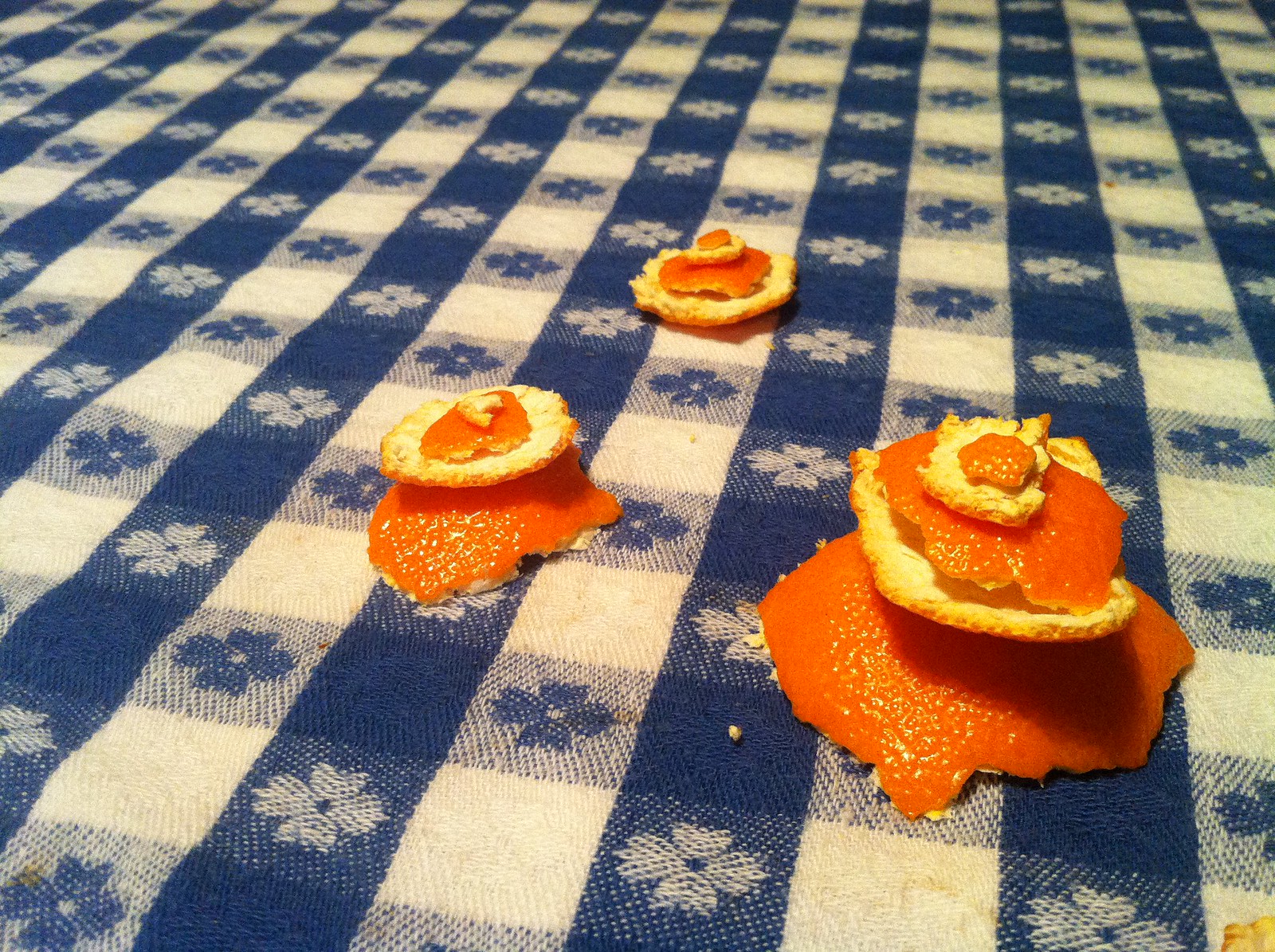This color photograph, shot indoors at an angle, captures a detailed scene of a white, light blue, and dark blue plaid tablecloth adorned with alternating flower patterns. The thin, crisscross tablecloth features blue lines with white flowers and white lines with blue flowers. Positioned on the tablecloth are three meticulously arranged groups of bright orange peels, forming a triangular formation. The largest group, situated at the bottom right, has a towering structure of five peels, starting with a large, downward-facing peel and topped with progressively smaller pieces. To the upper left, a slightly smaller group consists of four stacked peels. The smallest group at the center back begins with an upright peel creating a bowl, with three additional peels placed inside. Subtle water stains are visible on the tablecloth, adding to the textural detail of the scene.